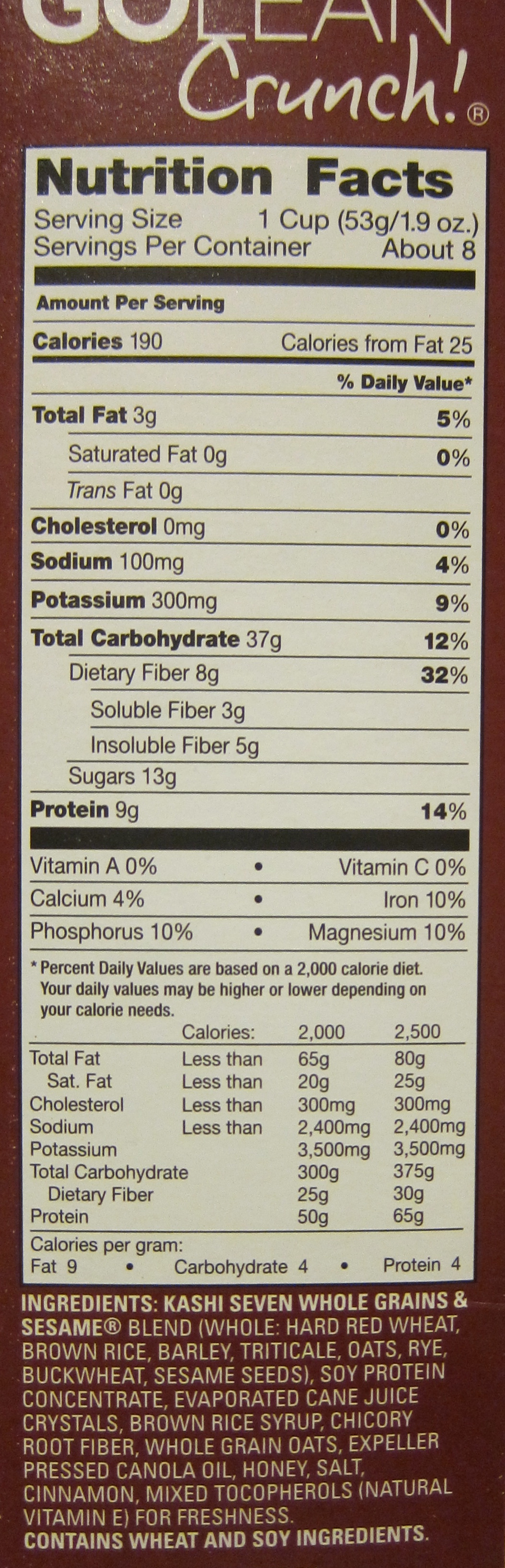The image displays the nutrition label on the side of a dark brown carton. At the top of the label, partially visible text includes a word starting with "G" followed by "Crunch." Below this, a large beige vertical rectangle prominently features "Nutrition Facts." This section provides detailed dietary information for a serving size of one cup (53 grams or 1.9 ounces), with approximately eight servings per container. Each serving contains 190 calories, with 25 calories from fat. The label breaks down nutritional components: 3 grams of total fat, low cholesterol, 100 milligrams of sodium, 300 milligrams of potassium, 37 grams of total carbohydrates, and the amounts of protein and various vitamins, listed beneath a bold black line. The bottom section of the label, with beige text on the dark brown background, details the ingredients, which include cashew, seven whole grains, a sesame blend, various whole grains like hard red wheat, brown rice, barley, oats, and rye, as well as buckwheat, sesame seeds, soy protein concentrate, evaporated cane juice crystals, brown rice syrup, chicory root fiber, whole grain oats, expeller-pressed canola oil, honey, salt, cinnamon, mixed tocopherols, and natural vitamin E for freshness. The label also notes that the product contains wheat and soy ingredients.